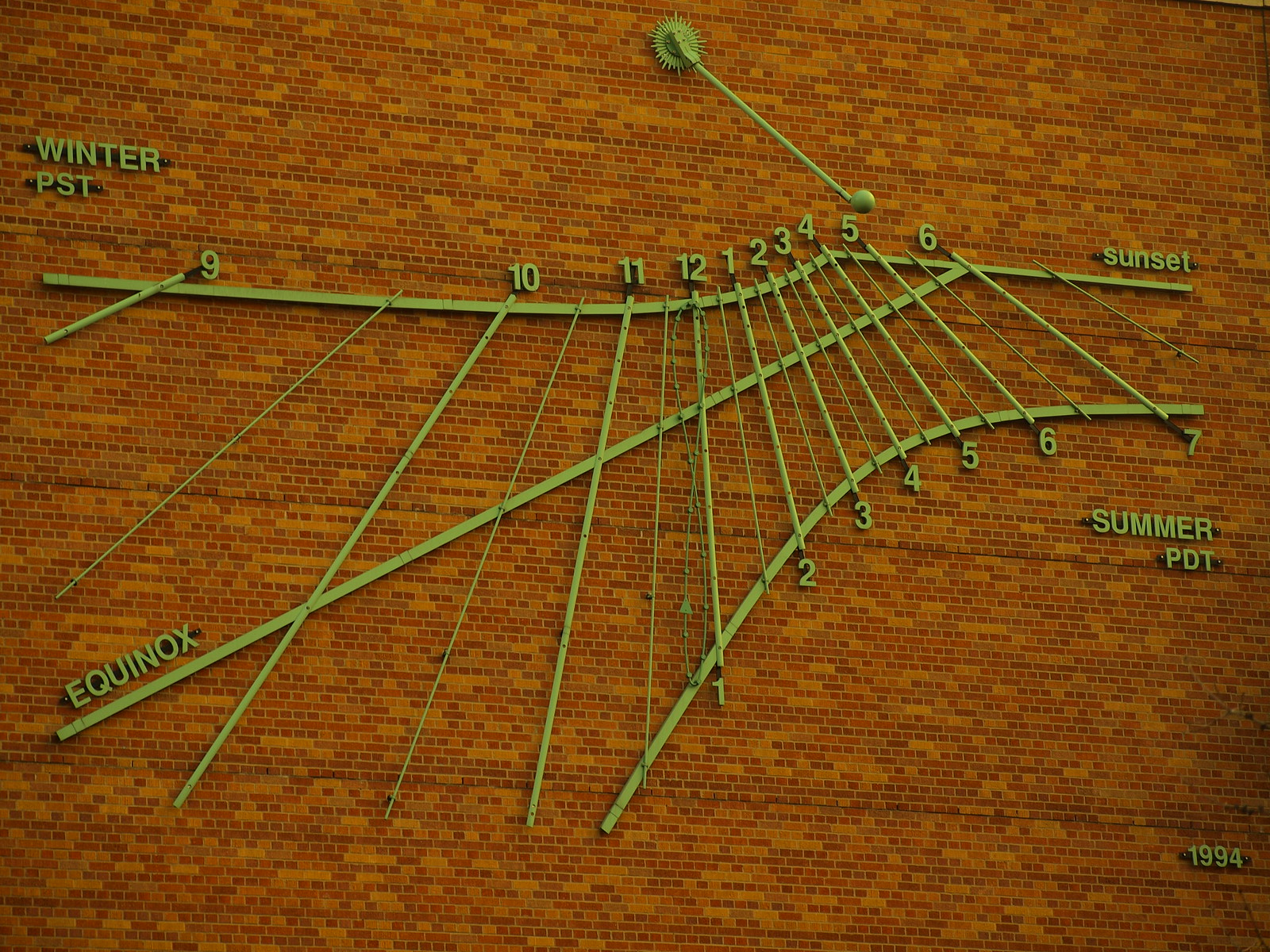The image features a brick wall background composed of various shades of bricks, ranging from dark to light. In the top left corner of the wall, there is a green patch with text indicating "winter" and "PST". On the bottom left, the word "equinox" is written and stretches diagonally to the top right corner, where "sunset" can be seen. "North" is labeled as "summer" located towards the very bottom right. Additionally, a line marked with the numbers 9, 10, 11, 12, 1, 2, 3, 4, 5, and 6 leads towards "sunset". There are multiple diagonal lines intersecting the image, contributing to a dynamic composition that spans from the bottom right corner and connects various points including the equinox and sunset annotations.